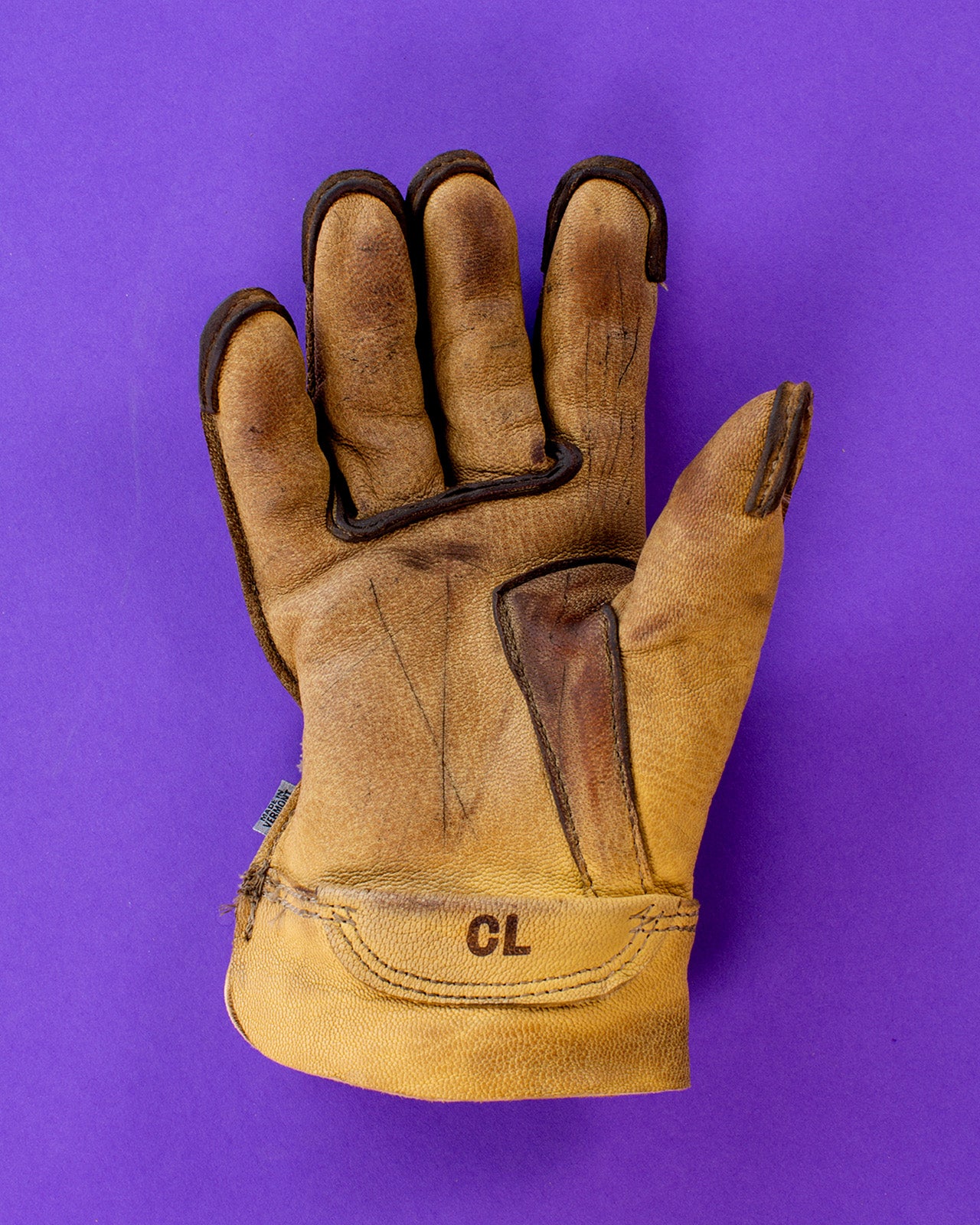The image features a detailed photo of a right-handed work glove, positioned against a vibrant purple backdrop. Captured from above, the glove is constructed from light brown leather and exhibits robust craftsmanship with its intricate, reinforced stitching. Thick stitching encircles each finger for added durability, extending between the middle and ring fingers, around the two middle fingers, and then between the first and middle fingers. A darker leather patch strengthens the thumb area, ensuring greater protection and longevity. Near the wrist, a stamped half-circle piece of leather displays the initials CL, indicating possible personalization. The glove, with its meticulous design and detailed reinforcements, suggests it is a high-quality item intended for rigorous use.